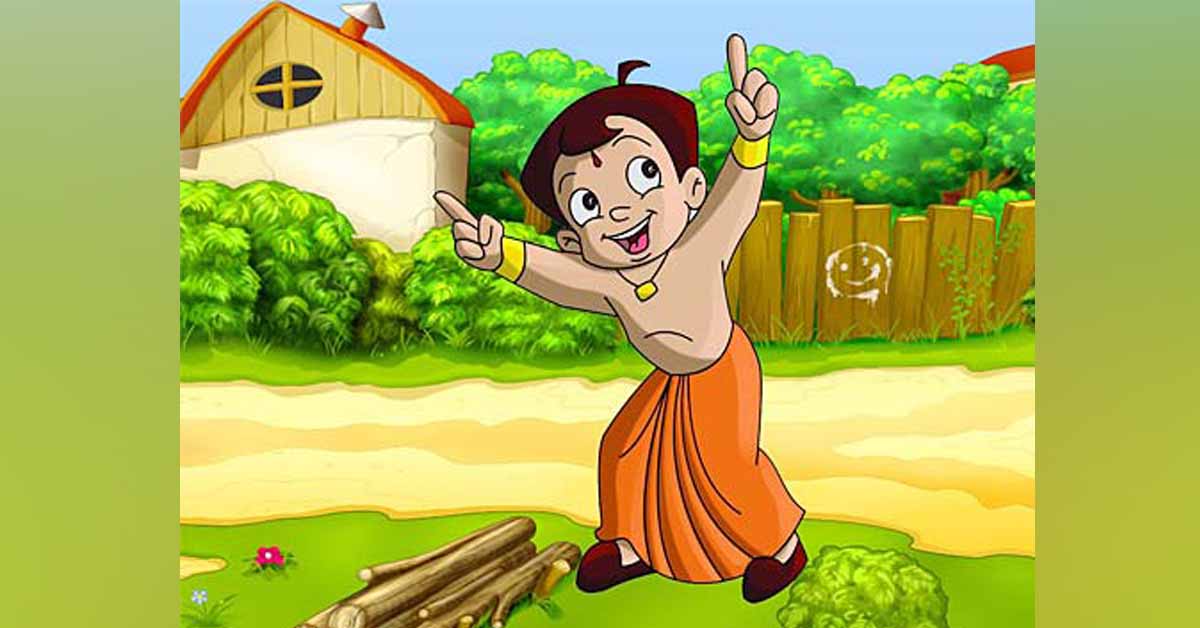This detailed illustration depicts a young cartoon boy, likely between eight to ten years old, standing outside. He has short brown hair with a distinctive strand sticking straight up like a rooster's tail feather, and a reddish teardrop mark between his eyes or on his forehead. The boy is shirtless and adorned with a gold necklace and gold wristbands. He wears an orange robe that extends to his feet, complemented by cranberry-colored slippers.

The setting appears to be a riverside yard or backyard, with the overall backdrop imbued in green hues. The boy stands on a patch of green grass, with his arms raised and index fingers pointing skyward. Behind him, there’s a wooden fence prominently featuring a white happy face drawing. To his left, there's a bundle of sticks and some flowers scattered on the ground. Further back, a dirt path leads towards a green-roofed house partially obscured by bushes. Additional trees are visible in the background, enhancing the lush, verdant ambiance of the scene.